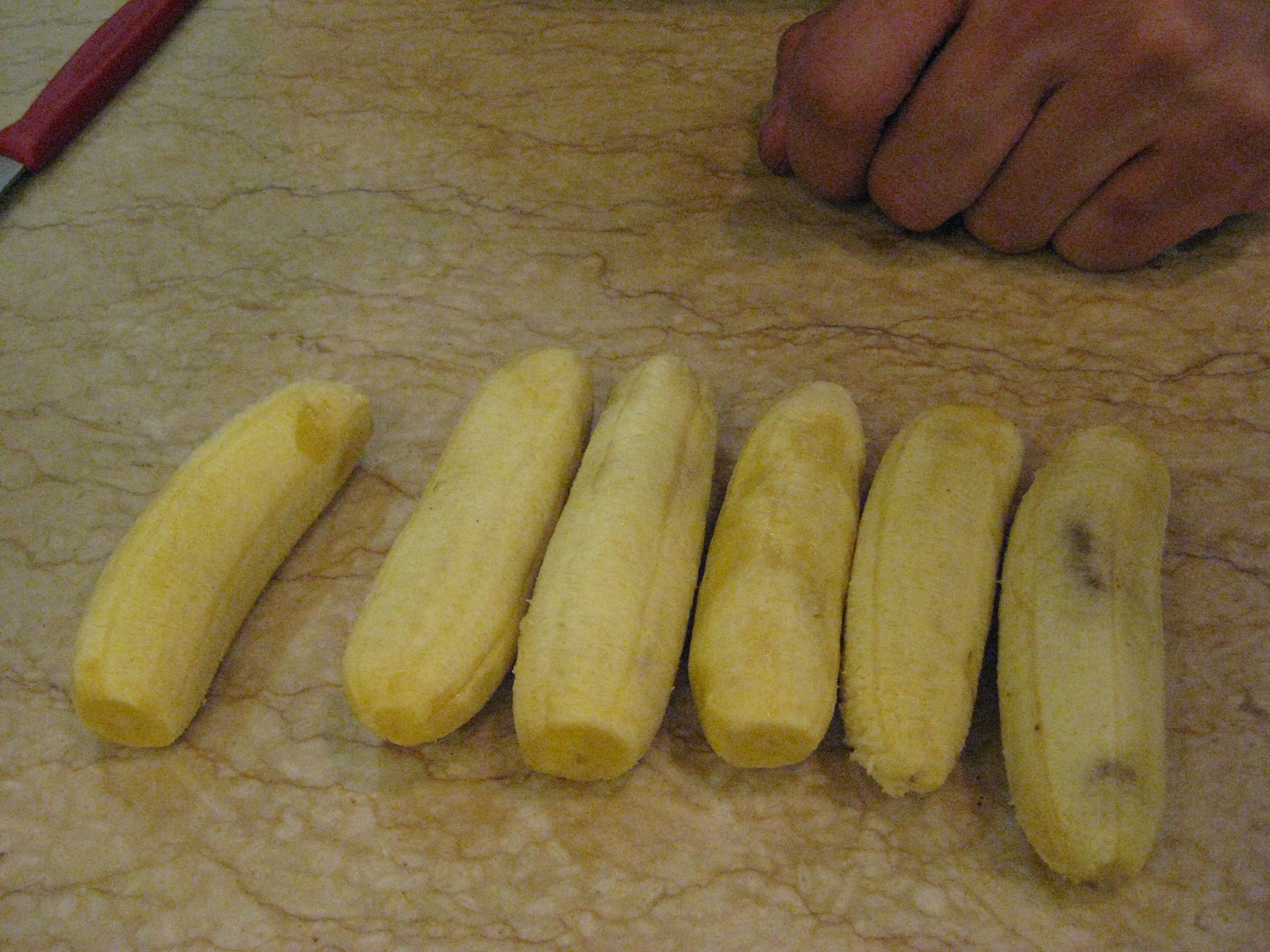The image features six peeled yellow bananas arranged in a line on a marble countertop, which has a cream base color with brown and orange marbled patterns. The first banana on the far left is slightly separated by about an inch from the rest, which are closely lined up from the second to the sixth on the right. Three of the bananas have one end cut off, while the other three are full length. The banana on the far right has two noticeable black spots. A person's hand, clenched into a fist, rests on the tabletop, hinting at recent activity of peeling or cutting the bananas. In the top left corner of the image, a red knife handle is visible, along with a small portion of the blade's edge.